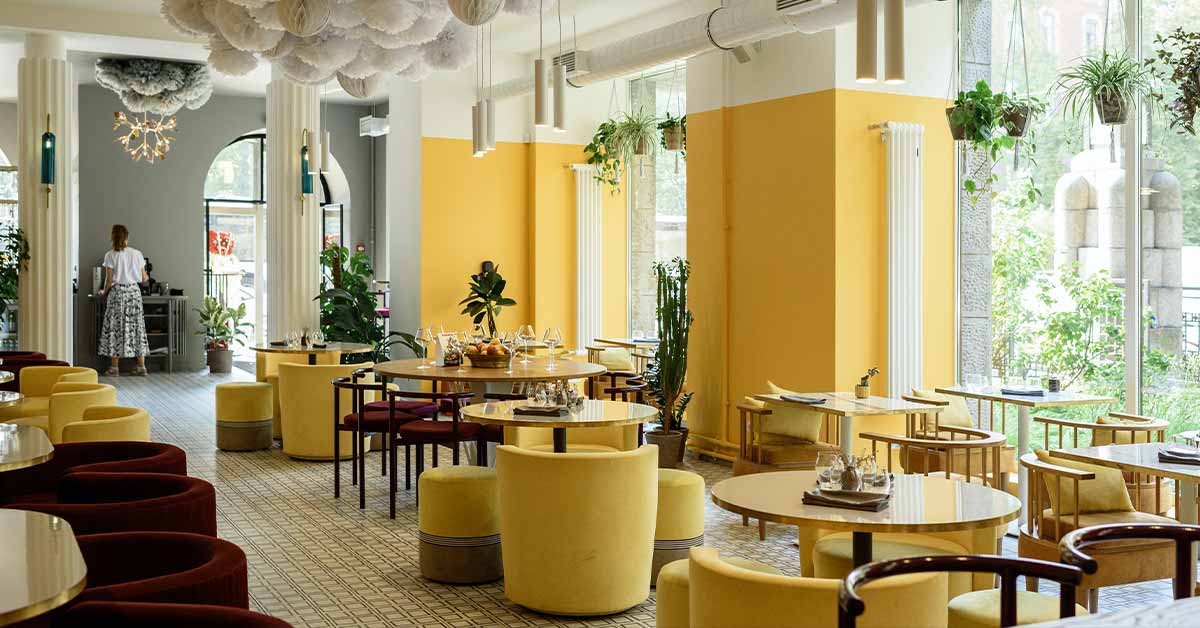The image portrays a bright and cheerful open-air dining room adorned with many round tables and vibrant yellow chairs. Dominating the center and right side of the room are these round tables, some accompanied by cylindrical seats without backrests and others with quarter-circle curved seats. To the left side, square tables take precedence, surrounded by slightly curved chairs that include armrests but lack backrests, predominantly colored in maroon and yellow tones. A lady dressed in a white top and a black and white skirt stands near a gray wall with a doorway, in front of shelves, towards the room's far left background. The room itself is bathed in light from tall, 10-foot windows spanning the room, framed by yellow and white walls that enhance the room’s bright atmosphere. These windows, adorned with hanging greenery, offer a view of lush plants outside, adding to the room's verdant and clean aesthetic.